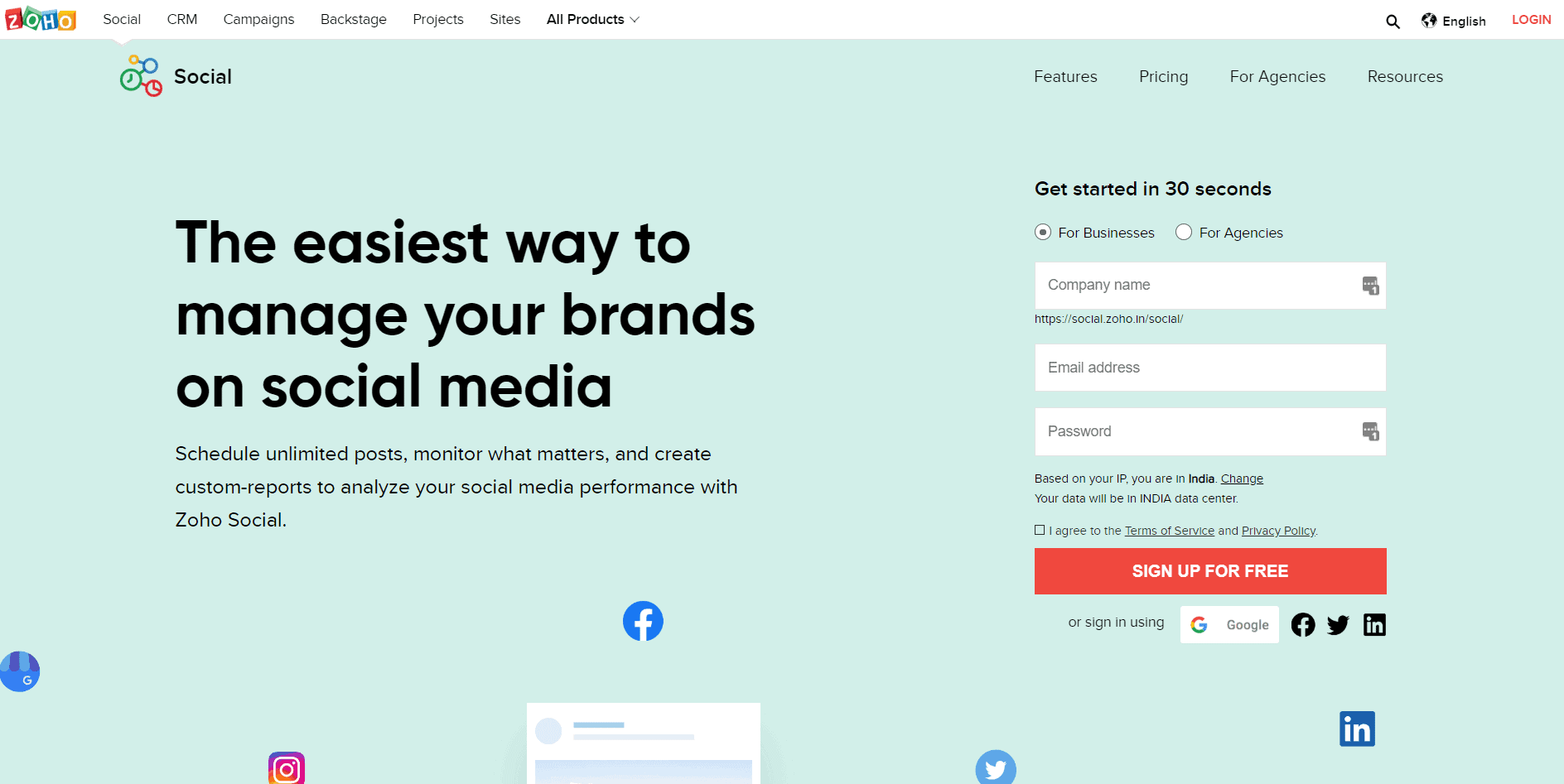Here is a cleaned-up and detailed caption for the image described:

---

The landing page for Zoho Social, a social media management platform, prominently displays various features and functionalities. The header reads "Zoho Social CRM Campaigns Backstage Project Site - All Products." Below this, an engaging tagline emphasizes, "The easiest way to manage your brands on social media." 

The page offers a brief overview of the platform's capabilities, including scheduling unlimited posts, monitoring key metrics, and creating custom reports to analyze social media performance. A standout message highlights the ease of getting started with Zoho Social, claiming users can begin in just 30 seconds.

There are dedicated fields for businesses and agencies to enter their company name and pertinent details. An example URL is provided: "http://social.zoho.in/social/," illustrating how the personalized social pages might look.

Additionally, the page prompts users to input their email and password. Based on the detected IP address, a notification informs users that their data will be stored in the local data center, in this case, India. A checkbox for agreeing to the "Terms and Services" and "Privacy Policy" is located near the bottom.

A prominent red button invites users to "Sign up for free," or alternatively, "Sign in using Google." There are also recognizable logos for Facebook, Twitter, and Instagram, displayed in small circular icons at the bottom of the page.